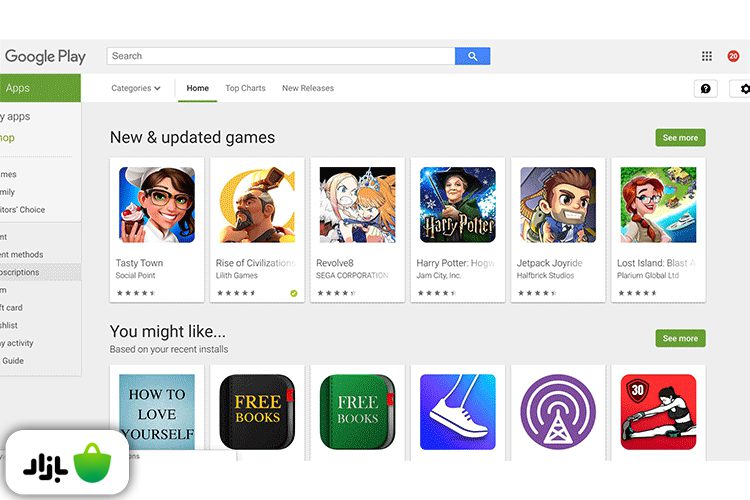This is a detailed screenshot of the Google Play website, capturing various elements and sections. At the very top, the prominent Google Play header is displayed followed by a search bar on the right, accompanied by a button featuring a magnifying glass icon for initiating searches.

Beneath the header, there's a section dedicated to "New and Updated Games." This section features a horizontal row of game icons, each enclosed in a rectangular box displaying an illustration and the game’s title. The games, listed from left to right, include:

1. **Tasty Town**
2. **Rise of Civilization**
3. **Revolve 8**
4. **Harry Potter: Hogwarts** (with part of the title grayed out and unclear)
5. **Jet Pack Joyride**
6. **Lost Island: Blast Something**

Below this section is another row of recommendations under the heading "You might like..." These suggestions are based on the user's recent installations. The icons in this row include:

1. **How to Love Yourself**
2. **Free Books** (depicted with a black background)
3. **Free Books** (another one, but with a green background)
4. An icon featuring the illustration of a leg in sneakers
5. An icon resembling a radio tower emitting signals
6. An icon showing a woman stretching, likely representing an exercise or fitness app.